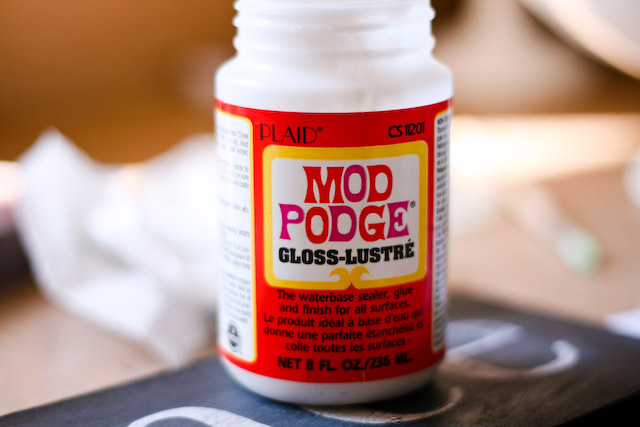The image features a prominently centered bottle of Mod Podge, captured with professional clarity against a blurred background, likely shot with a high-quality camera. In the background, there appears to be a white napkin or piece of fabric, partially obscuring other desk items, while the bottle rests on a brown wooden surface featuring partially visible white letters "C" and "E."

The Mod Podge bottle itself is a white container with a distinctive red label. The label includes a prominent yellow border and a white text area that reads "Mod Podge" in a 1960s psychedelic-style font. The product name is creatively stylized, with "MOD" in red and "Podge" mixing red and pink hues. Below the main text, it states "Gloss Lustre" in black letters.

Further down, the label adds in black text, "the water-based sealer, glue, and finish for all surfaces," with a corresponding French translation. Additional details include the identifier "Plaid" and what seems to be a product code, "CS11201". The bottle specifies it contains 8 fluid ounces of the product. This close-up shot appears to be capturing the bottle as part of an ongoing art project.